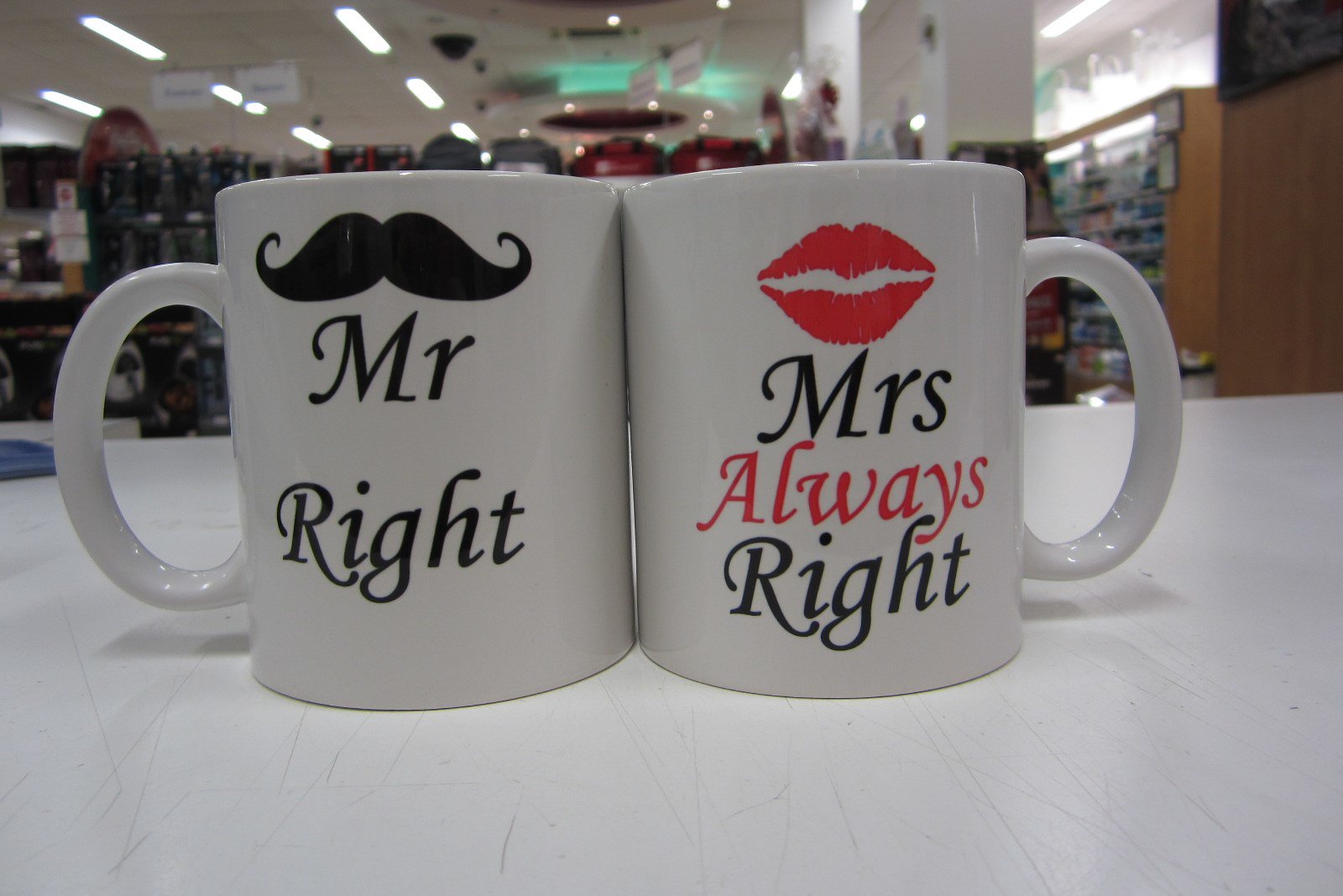This is a color photograph in landscape orientation featuring two white coffee mugs positioned side by side on a white table. The mugs, identical in shape and style, have their handles facing outward, with the left mug's handle pointing to the left and the right mug's handle pointing to the right. The mugs meet at the center, creating a sense of unity. On the left mug, the text "Mr. Right" is printed in bold black italic script, accompanied by an image of a black mustache above the text. The right mug displays the text "Mrs. Always Right," with "Mrs." and "Right" in black letters and "Always" in red letters, topped by a red lip imprint. The background features the blurry interior of a store, discernible through signs hanging from the ceiling and various merchandise on the shelves. The scene is illuminated by inset ceiling lights, enhancing the representational realism of the photograph.